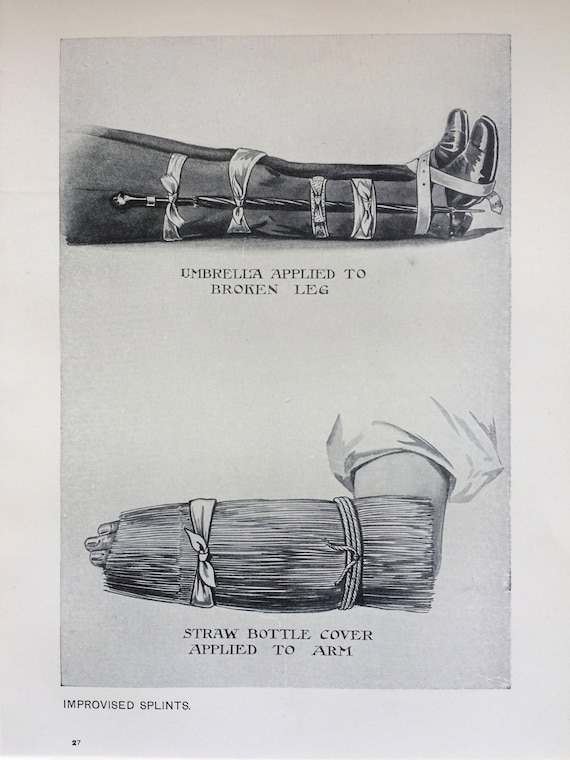This black-and-white image appears to be a page from an old book or magazine, possibly from the early 20th century, presented on light gray, aged paper. It features two hand-drawn diagrams demonstrating improvised splints. The page is numbered 27 and titled in black uppercase letters, "IMPROVISED SPLINTS."

The upper illustration depicts a person's lower legs, richly detailed with dark pants and shiny leather shoes. An umbrella, described as having a black handle and pointed tip, is tied to the right leg from thigh to ankle using fabric straps. The text beneath this drawing reads, "Umbrella applied to broken leg," illustrating an emergency splint made from an umbrella.

The lower illustration shows an improvised splint for an arm, wrapped in what appears to be a straw bottle cover, held together with ropes and fabric ribbons. The drawing is labeled, "Straw bottle cover applied to arm," indicating a makeshift cast made from straw to stabilize the arm. Overall, the page offers a fascinating glimpse into historical first-aid techniques using readily available materials.